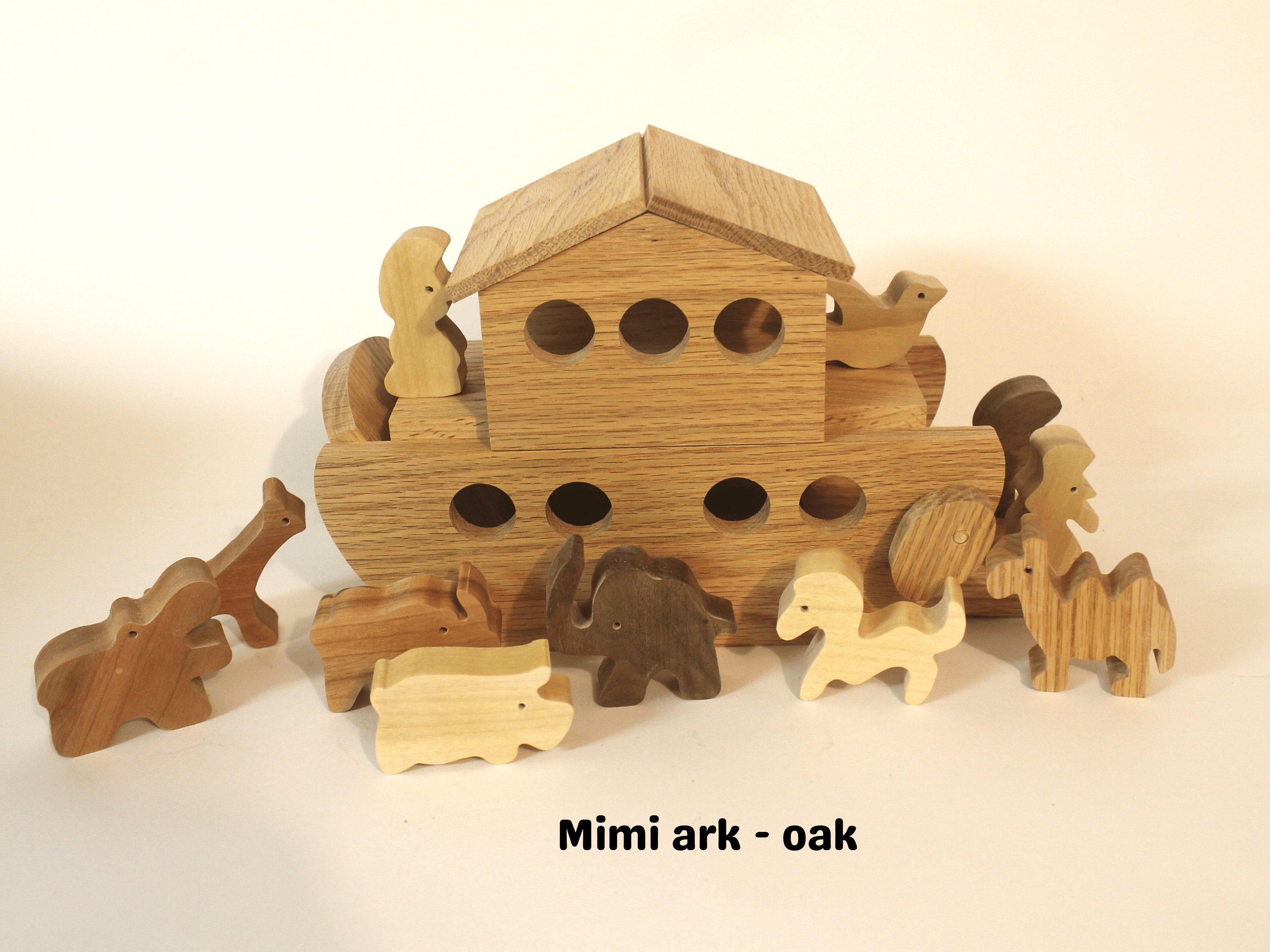Displayed on a tan table is an entirely wooden toy set of Noah's Ark. The ark itself is the focal point of the image, comprising two slanting roofs that appear to be functional for storage, given the visible openings. The main body of the ark features four circular windows on the bottom layer and three on the upper layer. At the forefront of the ark are seven finely crafted wooden animals, including a dark elephant, a light-colored horse, a two-humped camel, a low rhinoceros, a giraffe, and a hippopotamus in varying shades of wood. Additionally present are a cutout figure of Noah behind the ark and a figure of the dove in front. The base is inscribed with "Mimi Ark/Oak." The ark evokes an engaging children's project, potential as both a plaything and an educational tool, reflecting different hues of pine wood and emphasizing its hand-carved details.